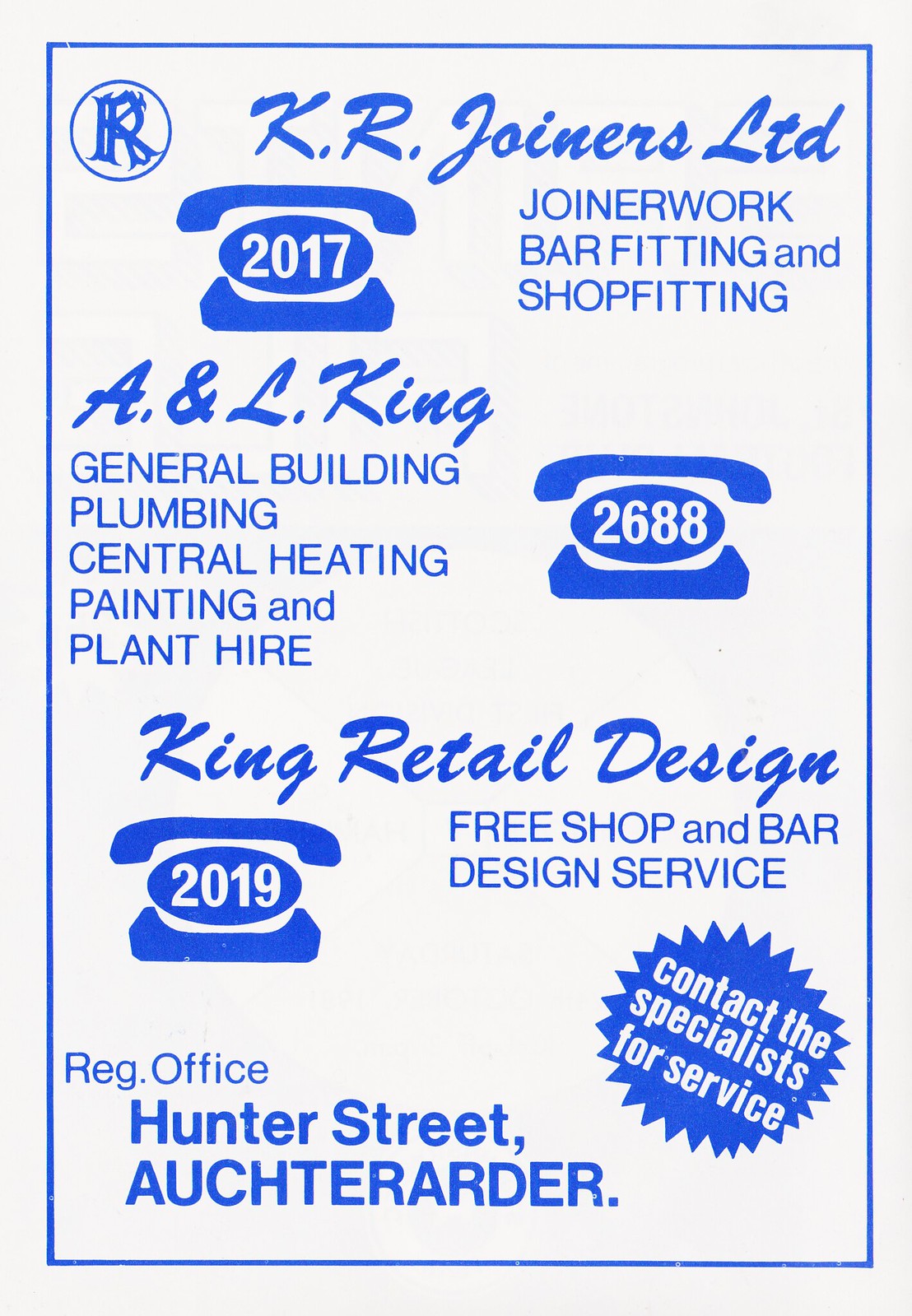This is a vintage, full-page, rectangular advertisement, likely from an official program or magazine, characterized by its distinct blue ink on a white background and designed in a portrait orientation. The top section of the flyer features a circular logo with the letters "R" and "K" inscribed, followed by the headline "K.R. Joiners Limited" in an italicized, almost cursive font. Directly beneath the headline, the flyer advertises services such as "Joiner Work, Bar Fitting, and Shop Fitting," all in uppercase letters except for "and." 

Adjacent to this text on the left side is a blue telephone icon displaying the number 2017. Below this section, on the left side, it states "A & L King General Building, Plumbing, Central Heating, Painting, and Plant Hire." Next to this text, on the right side, is another telephone icon showing the number 2688. 

The bottom portion of the flyer reads "King Retail Design," followed by "Free Shop and Bar Design Service," with a telephone icon to the left displaying the number 2019. Further down, the text "Registered Office: Hunter Street, Auchterarder" is located at the bottom left corner. Finally, in the bottom right corner, there is a spiked, asterisk-like logo in blue, with the accompanying text: "Contact us, specialists for service," in white.